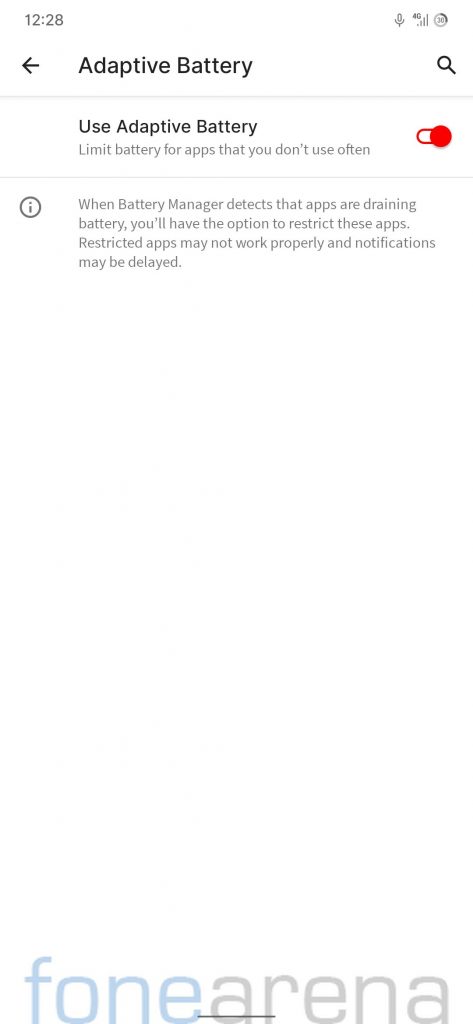The screenshot appears to be from a mobile phone displaying a settings page, specifically focusing on battery management options. Dominating the screen is a considerable portion of white space, contributing to a perceived elongation of the overall image.

At the very top-left corner, the screen shows a timestamp of "12.28" and several small mobile icons, including a "4G" indicator, are aligned to the right-hand side. Below this cluster, the title "Adaptive Battery" is prominently written in black, flanked by a back arrow on the left and a small search icon on the right. Directly underneath this title is a subtle grey horizontal line.

The section following this line contains a toggle option labeled "Use Adaptive Battery," which displays a red slider set to "on." Beneath this, smaller text advises, "Limit battery for apps that you don't use often." Another thin horizontal line demarcates this section from the subsequent informational text.

A small circle containing the letter "i" (info icon) is positioned to the left of a paragraph stating: "When Battery detects that apps are draining battery, you'll have the option to restrict these apps. Restricted apps may not work properly, and notifications may be delayed."

The remainder of the image comprises approximately 80% blank space, which creates an unusual and overly tall appearance for a typical phone screenshot. At the very base of the image, a watermark for a website named "Phone Arena" is present. The word "Phone" is stylized as "F-O-N-E" in blue, and "Arena" is rendered in grey.